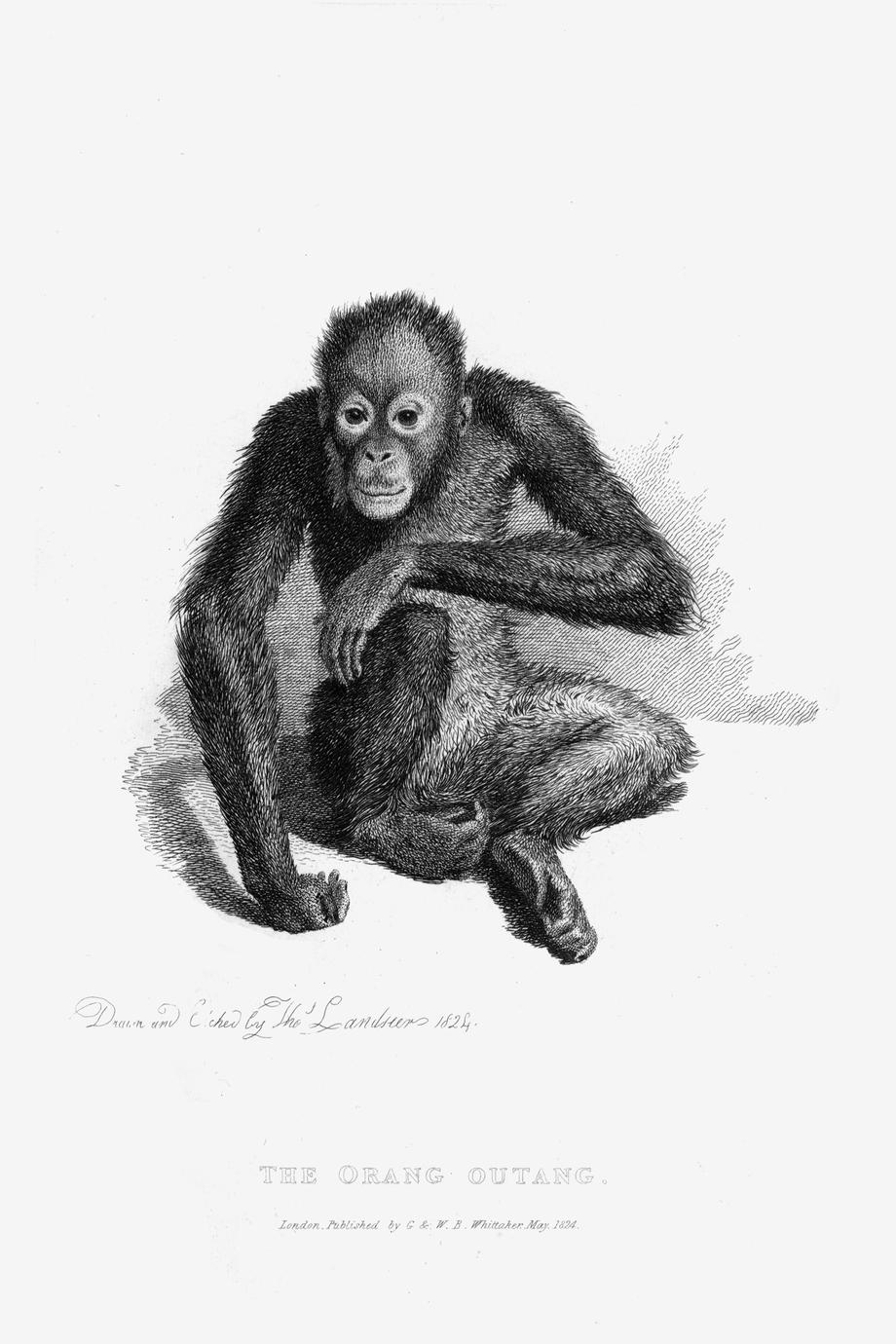This vintage pen and ink drawing, likely published in London around 1824, depicts an orangutan labeled "Orang-Otang" in three separate words at the bottom. The detailed illustration, composed of many short pen strokes, portrays a presumably juvenile orangutan sitting on the ground. One of its legs is bent with the knee drawn up towards its chest, while the other leg is tucked beneath it, giving a semi-crossed appearance. One arm rests on the ground with its fingers curled up, and the other arm is bent at a right angle, with its hand resting on the knee. The orangutan faces forward with open eyes and light rings around them, displaying a neutral expression. The background features a gray shadow, contrasting with the white backdrop. The intricate drawing highlights the thin, long limbs and fuzzy texture of the orangutan's fur.